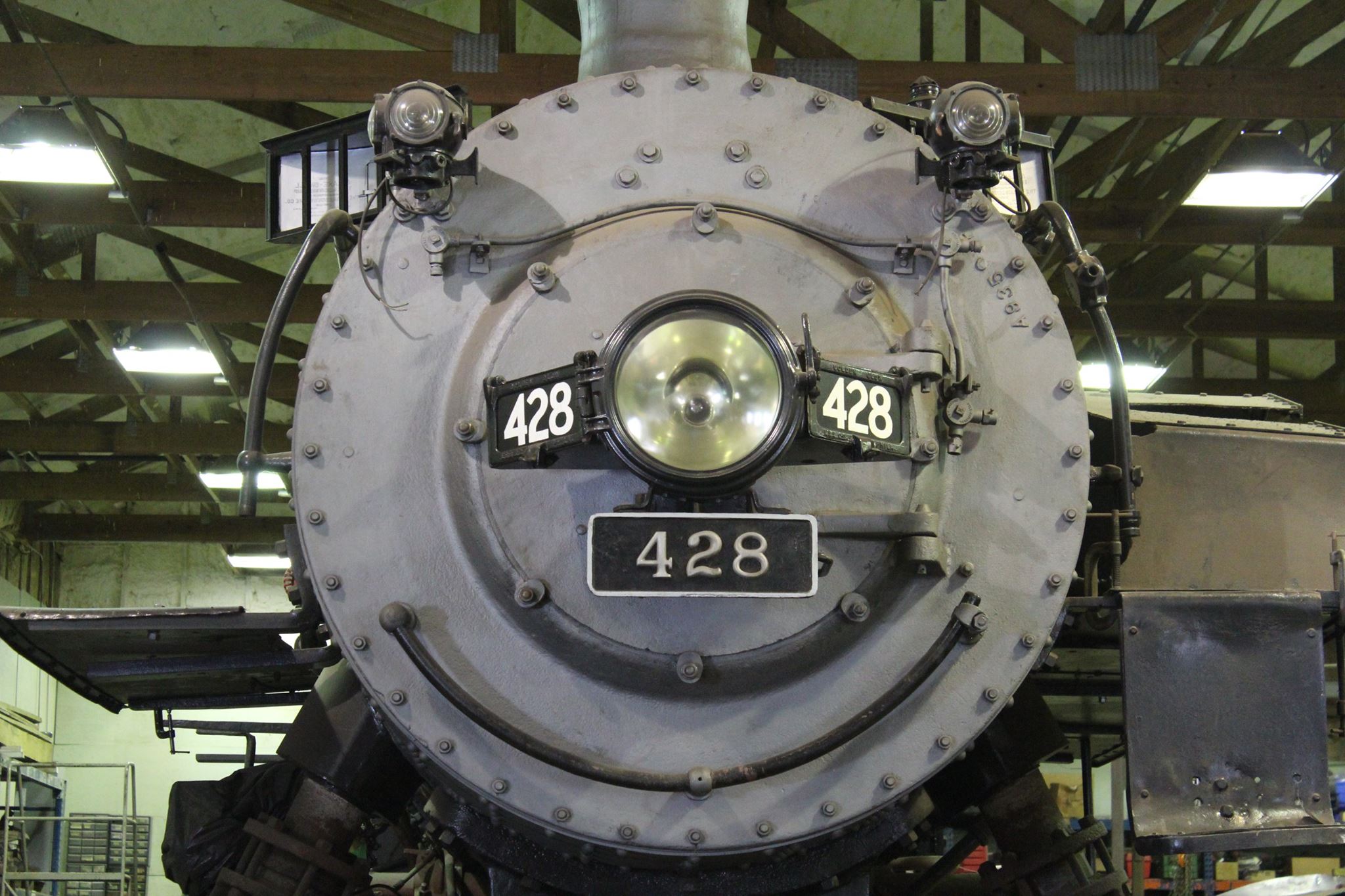This detailed close-up photograph showcases the front of a vintage steam engine train, drawing a parallel to a smiling face. Dominating the scene is a large, gray circular boiler face, studded with numerous rivets and bolts. At the center of this circle is a prominent headlight, flanked by two smaller lights positioned at approximately the 1 and 11 o'clock marks, giving it a face-like appearance reminiscent of "Thomas the Train."

Three sets of the numbers "428" feature prominently: two are displayed on metal flaps angled at 45 degrees to the left and right of the central headlight, while the third set is emblazoned on a plaque positioned below the headlight, bordered by a white outline. Beneath the plaque, a steel component arcs upwards, enhancing the face-like visage of the train front.

The background reveals an interior setting, likely a barn, warehouse, or repair shop, where the train is undergoing maintenance. Wooden beams and trusses support the ceiling, with additional metal reinforcements and nails lending structural stability. Fluorescent lights are strung across the ceiling, illuminating the scene. To the right of the train, assorted metal pieces hint at repair activities, while tools and toolboxes are arrayed against a grayish-green wall on the left. The ambiance suggests a meticulous and industrious atmosphere enveloping this historic steam locomotive.